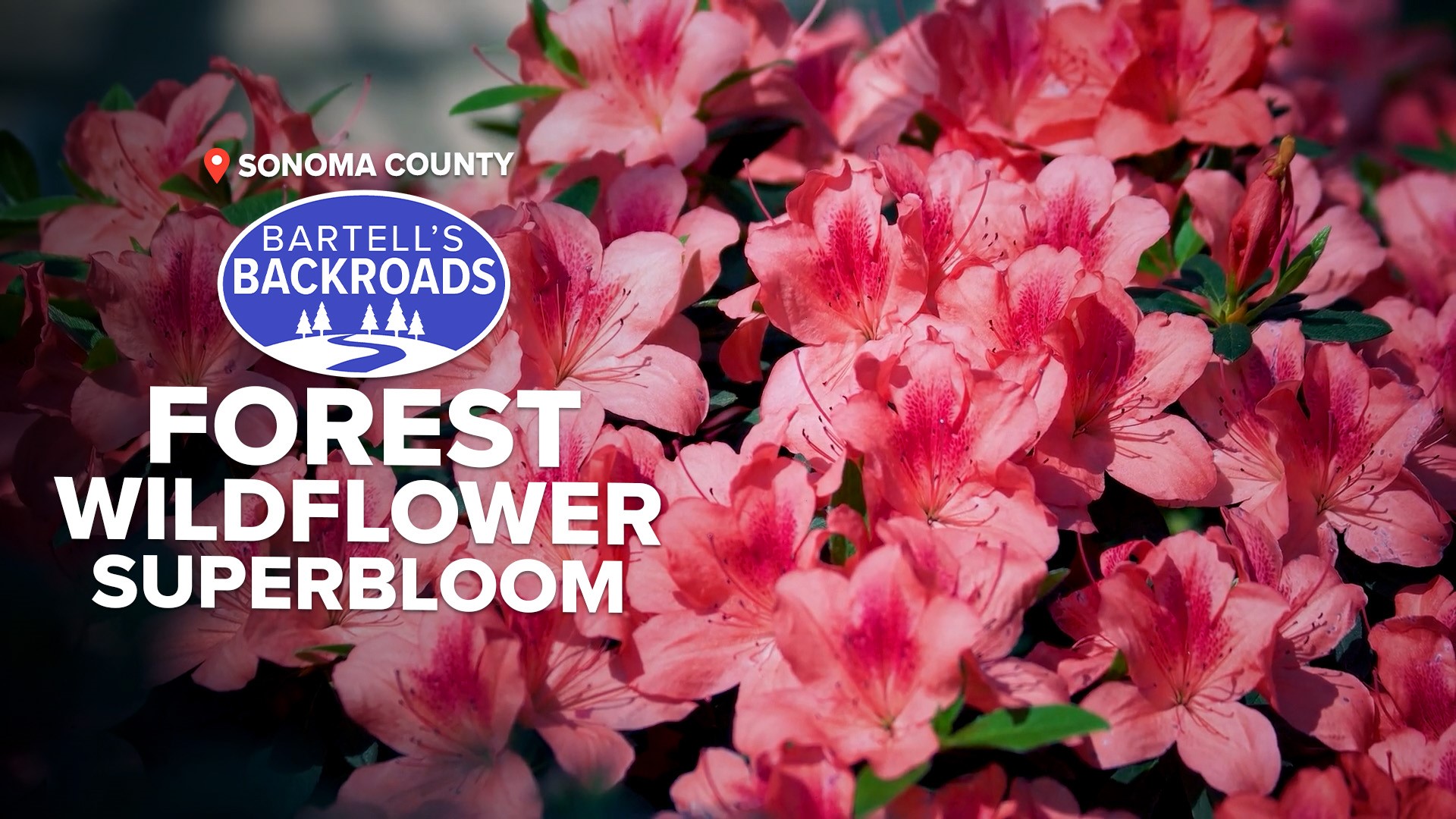This beautifully shaded and faded photograph captures an up-close view of vibrant flamingo-pink hibiscus flowers set against sparse green leaves. The image stretches from the left to right side, showcasing the delicate and striking blooms. On the left side, white text reads "Sonoma County" with a red marker symbol next to it, followed by a distinctive ovoid logo. The blue and white logo, with text that reads "Bartels Backroads," depicts a small road ascending a hill topped with pine trees. Beneath this logo, further text announces "Forest Wildflower Superbloom," indicating this poster promotes the rare and stunning wildflower display in Sonoma County. The overall composition, with its pink flowers tinged with red and the subtle greenery, makes for a visually pleasing and detailed advertisement.